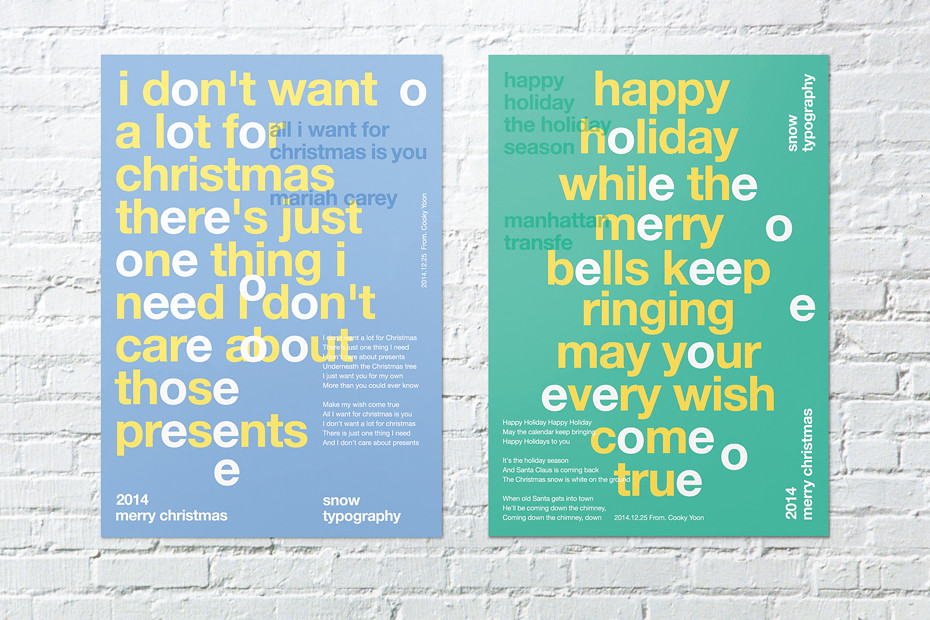This image features two festive Christmas posters mounted side by side on a white brick wall. The poster on the left has a light blue background and is adorned with a combination of yellow and white text, where all the O's and E's are highlighted in white. The poster reads, "I don't want a lot for Christmas, there's just one thing I need. I don't care about those presents." In a playful overlapping manner, white text further declares, "All I want for Christmas is you, Mariah Carey." Additionally, the lower left corner states "2014 Merry Christmas," and the lower right corner credits "Snow Typography."

The poster on the right features a green background with similarly styled yellow and white text, where all the O's and E's are also white. It reads, "Happy holiday while the merry bells keep ringing, may your every wish come true." The upper left corner reads, "Happy Holidays, the holiday season, Manhattan Transfer." In the lower left corner, there are more lyrics in white text, and the lower right corner again mentions "2014 Merry Christmas." Both posters contribute to a festive and harmonious holiday theme through their coordinated design elements and joyful Christmas messages.